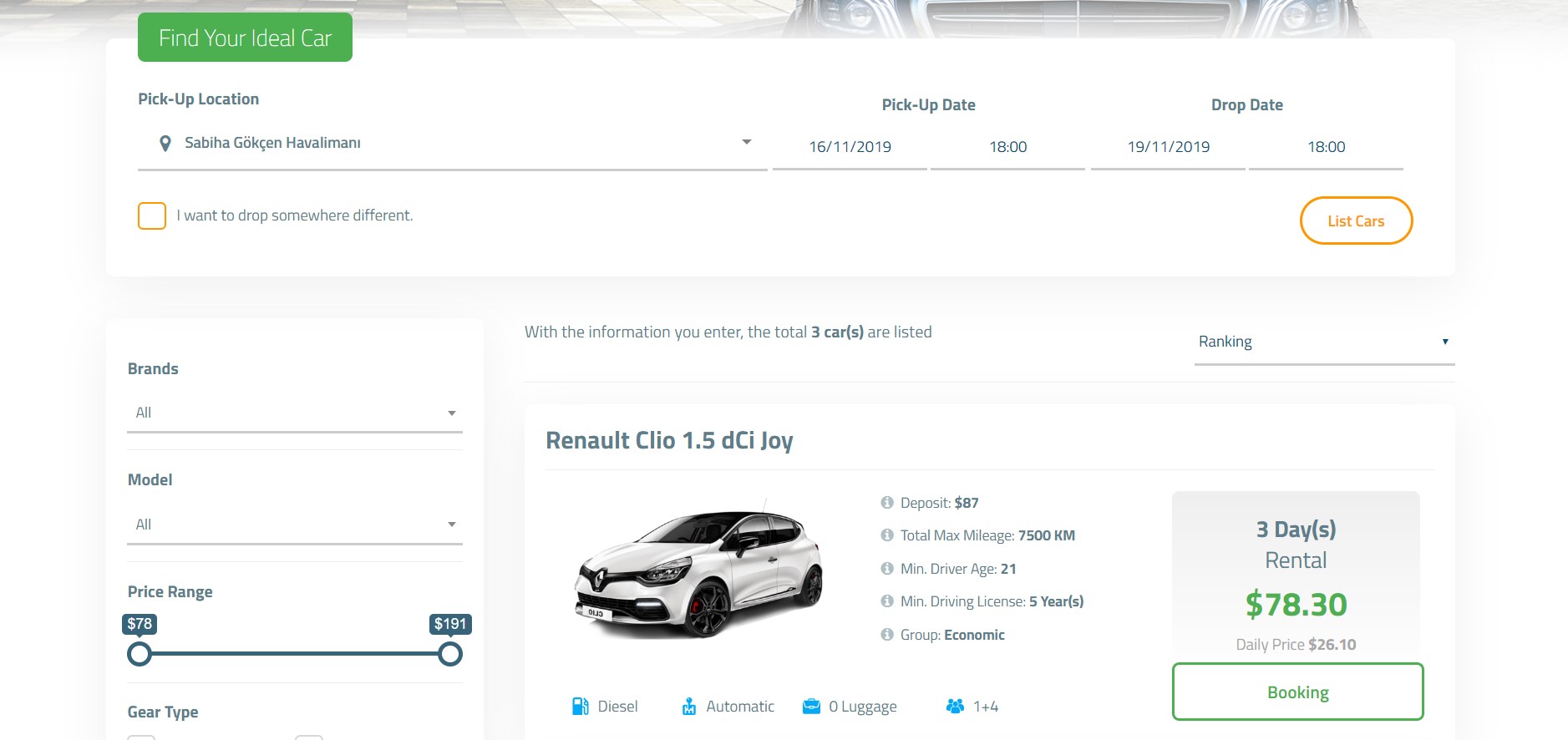This screenshot from a computer display shows a car rental selection page. At the very top left corner, a small green box reads "Find your ideal car." Just below, there's a section for selecting the pickup location, marked with a city name and a location icon, accompanied by a drop-down arrow for additional options. The text also reveals a specified pickup date of 16-11-2019 at 18:00 hours.

Beside the pickup date field, there's also a drop-off date field, indicating a return date of 19-11-2019 at 18:00 hours. On the left-hand side below these fields, an orange box offers an option to "Drop somewhere different," while the far right side features a "List cars" button.

In the main panel below these options, the left section provides filters for brands, model, and price range, with "All" listed under both brands and models, and a price range specified from $78 to $191. Below these filters, there is an option to select the gear type. 

To the right of these filters, text indicates that a total of three cars match the entered criteria. An option for ranking, with a drop-down arrow, is also available on this panel.

The car listed within this panel is a Renault Clio 1.5 DCI Joy, described as a white vehicle with black windows and black rims. The rental details include a deposit amount of $87, a maximum mileage limit of 7,500 kilometers, a minimum driver age of 21, a minimum driving license requirement of five years, and a classification of 'Economic.' 

The rental cost for a three-day period totals $78.30, with a daily rate of $26.10. Below this information, a booking option is prominently displayed.